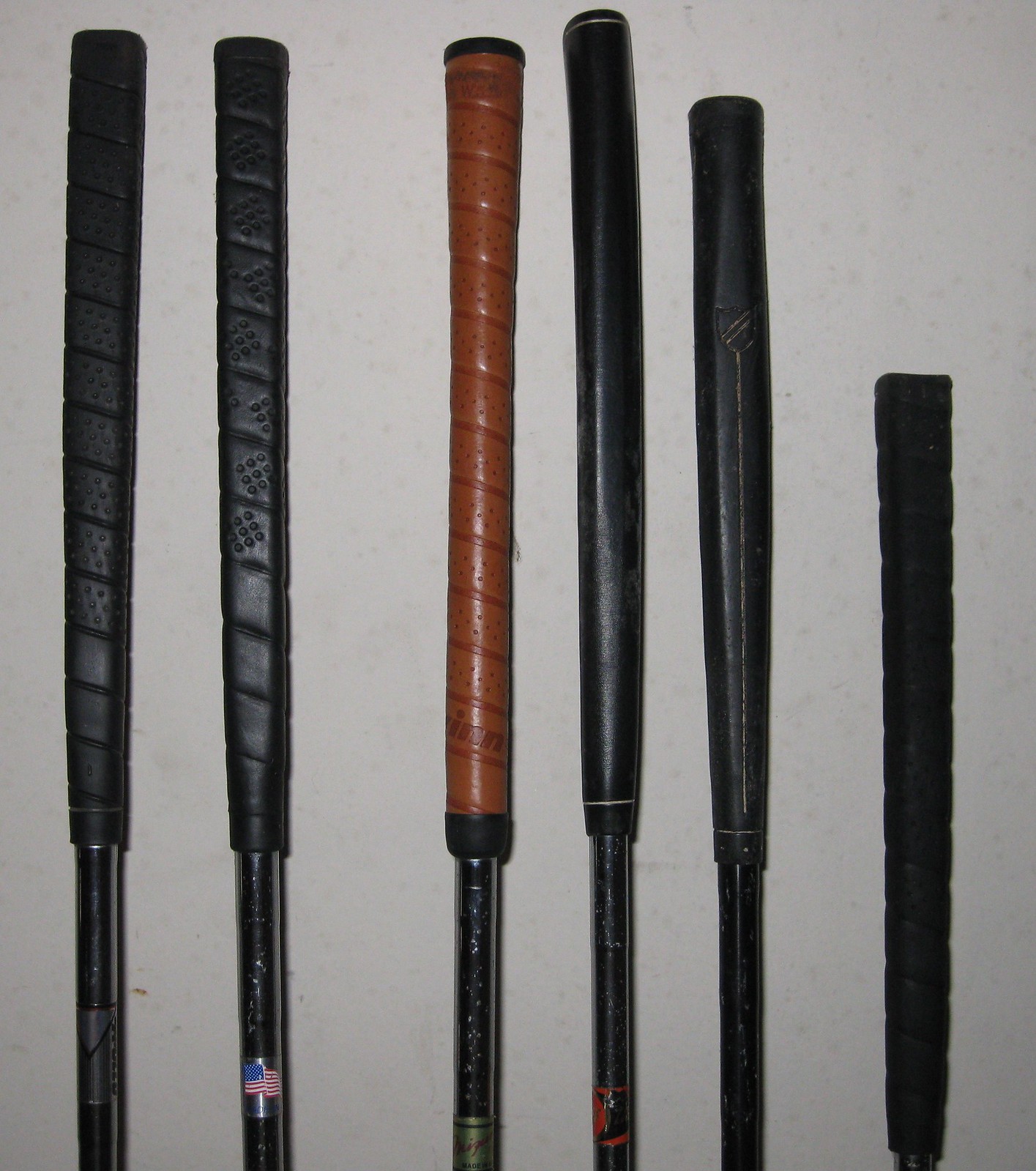This photograph features a collection of six vertically positioned, black metal cylindrical objects, potentially tools or athletic instruments, laying against a white background that appears slightly lighter in the middle. The objects are outfitted with grips, primarily black, which could be made of plastic, leather, or a similar material for a textured, grippable surface. From left to right: the first object is entirely black; the second is also black but adorned with an American flag decal; the third has a black body with a green sticker towards the base and a brown grip; the fourth presents a black exterior with a small red and black sticker; and both the fifth and sixth objects are entirely black with no visible markings.